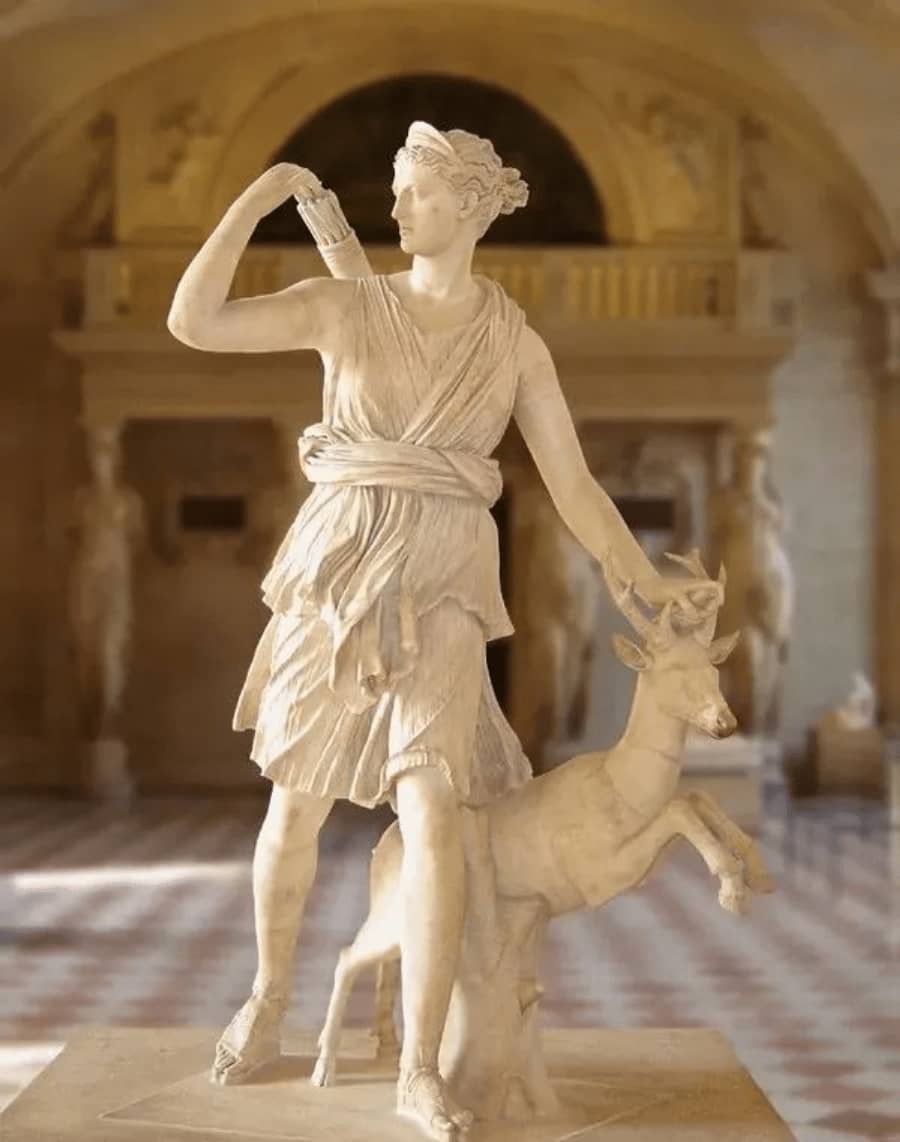This photograph captures a life-sized marble statue of Diana the Huntress, situated elegantly within a museum. The statue portrays Diana, the Roman goddess of hunting, adorned in a tunic that flows to her knees, cinched with a belted sash. Her hair is styled in a small ponytail, topped with a subdued crown. Diana is depicted in mid-motion, shifting her weight forward as she reaches back with her right hand to draw an arrow from her quiver. Her left hand holds a small stag, gripping its antlers and lifting it so that it stands on its hind legs. The marble figure exudes a sense of dynamic grace and readiness, perfectly embodying the classic Greco-Roman style. In the blurred background, other sculptures are faintly visible, including two female figures serving as pillars supporting an overhang, enhancing the museum's majestic ambiance. The pedestal on which Diana stands features a distinct diamond emblem, further adding to the statue's intricate details and the scene’s overall elegance.